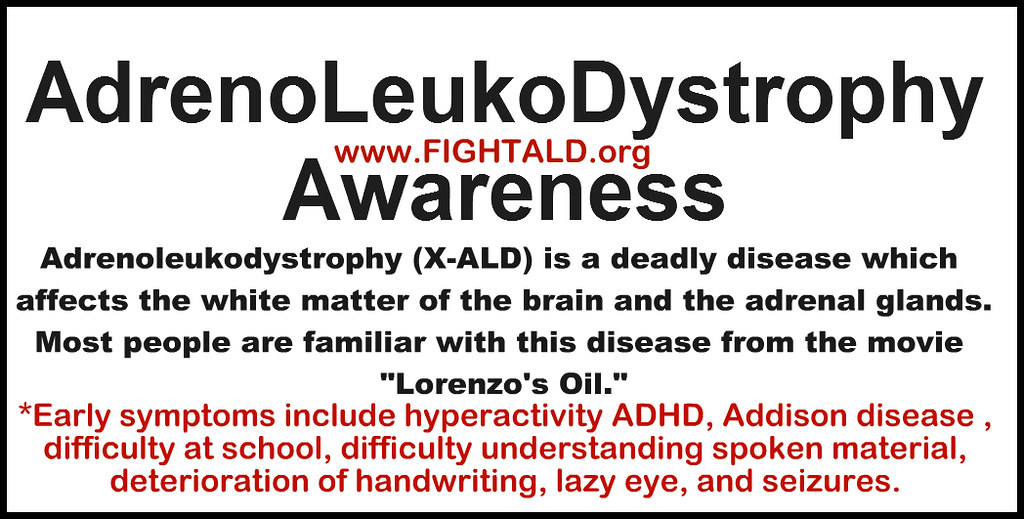The image features a large white rectangle with a prominent black border. At the top, in bold black text, it reads "Adrenoleukodystrophy." Directly below in striking red text is the web address "www.fightald.org." Further down, in smaller black text, it continues with "Awareness." The subsequent smaller black text reads: "Adrenoleukodystrophy (X-ALD) is a deadly disease which affects the white matter of the brain and the adrenal glands. Most people are familiar with this disease from the movie 'Lorenzo's Oil'." Following this, in red text accompanied by an asterisk symbol, it lists early symptoms: "Hyperactivity, ADHD, Addison's disease, difficulty at school, difficulty understanding spoken material, deterioration of handwriting, lazy eye, and seizures." The detailed layout is carefully designed to emphasize the critical information about the disease and directs viewers to the website www.fightald.org for more awareness.